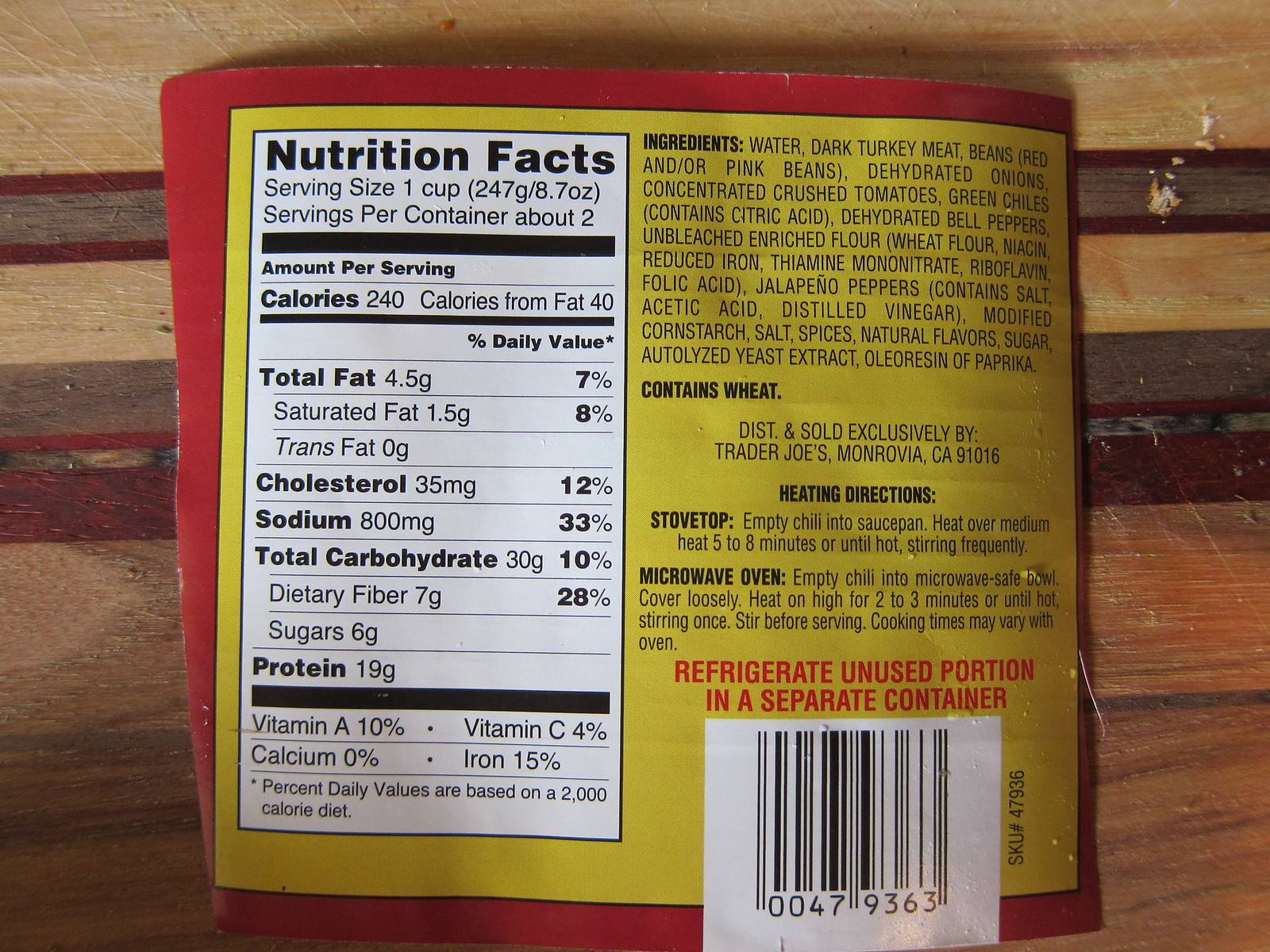This photograph captures the back of a nutrition label, clearly removed from its original packaging, now placed on a wooden cutting board with faint knife marks. The label features a red border and a yellow section with a thin black border, prominently displaying the nutrition facts in a white box with black text. The nutritional information reveals a serving size of one cup (247 grams or 8.7 oz), with approximately two servings per container. Each serving contains 240 calories, 40 of which are from fat. The breakdown includes 4.5 grams of total fat (7% daily value), 1.5 grams of saturated fat (8% daily value), 35 milligrams of cholesterol (12% daily value), 100 milligrams of sodium (33% daily value), 30 grams of total carbohydrates (10% daily value), 7 grams of dietary fiber (28% daily value), 6 grams of sugars, and 8 grams of protein. The vitamins and minerals listed are Vitamin A (10%), Vitamin C (4%), Calcium (0%), and Iron (15%). The label also outlines ingredients, including water, dark turkey meat, beans (red and/or pink), dehydrated onions, concentrated crushed tomatoes, green chilies, citric acid, dehydrated bell peppers, and unbleached enriched flour (wheat flour, niacin, reduced iron, thiamin, mononitrate, riboflavin, folic acid). Additionally, it contains jalapeno peppers (with salt, acetic acid, and distilled vinegar), modified cornstarch, salt, spices, natural flavors, sugar, hydrolyzed yeast extract, and oleoresin of paprika. Important storage instructions in bold red letters emphasize refrigerating unused portions in a separate container. The bottom of the label features a barcode and is entirely distributed and sold exclusively by Trader Joe's. The image suggests the label is from a chili product, confirmed by the heating instructions for both stovetop and microwave preparations.